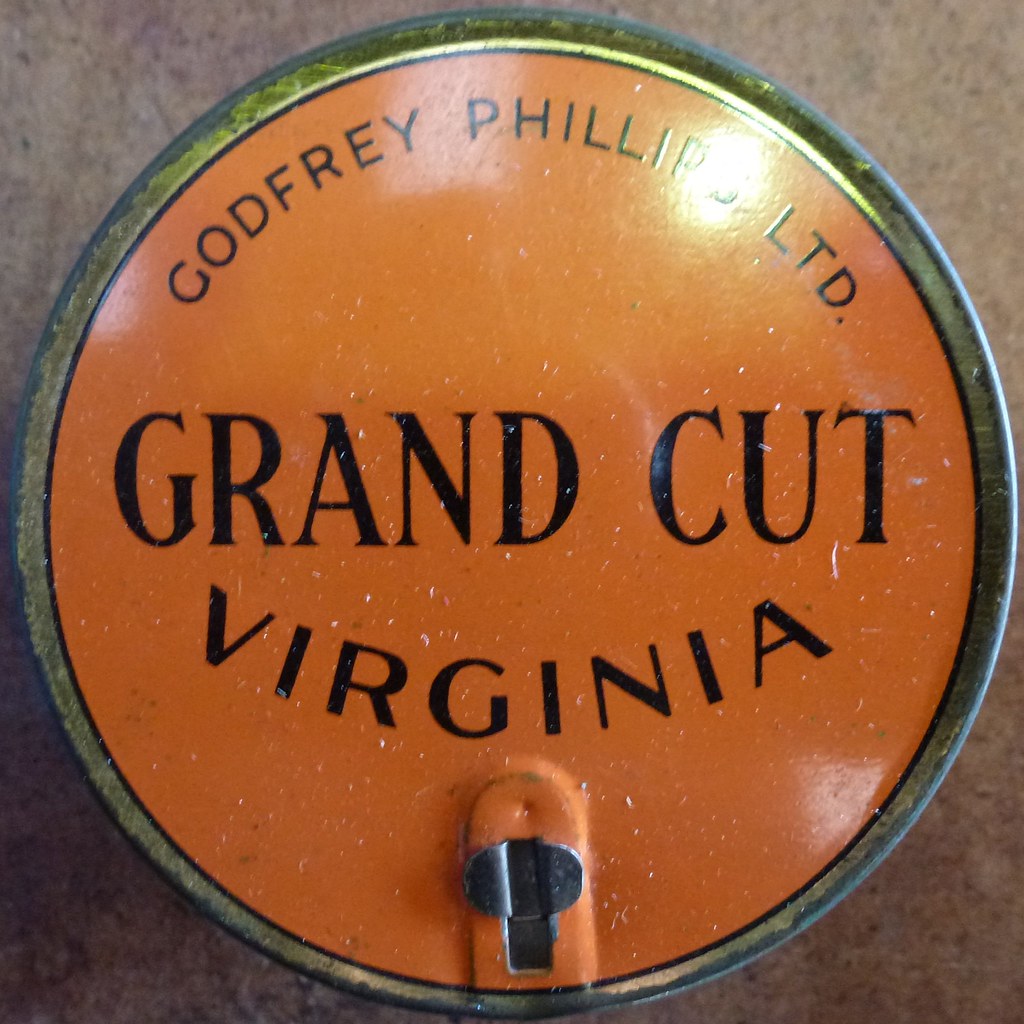This is a photograph taken directly from above, showing the top of a can resting on a brown, stone table. The can's cap is primarily orange with a green outer edge and a thin black border. Around the cap's top edge, it says "Godfrey Phillips Limited" in black text. Dominating the center, in bold black text, are the words "Grand Cut." Below this, in a curved, smile-like arrangement is the word "Virginia." At the bottom center of the cap, there's a small metal clip that presumably serves as the can's opening mechanism. The table surface has a granite-like appearance with a light brownish, reddish color.